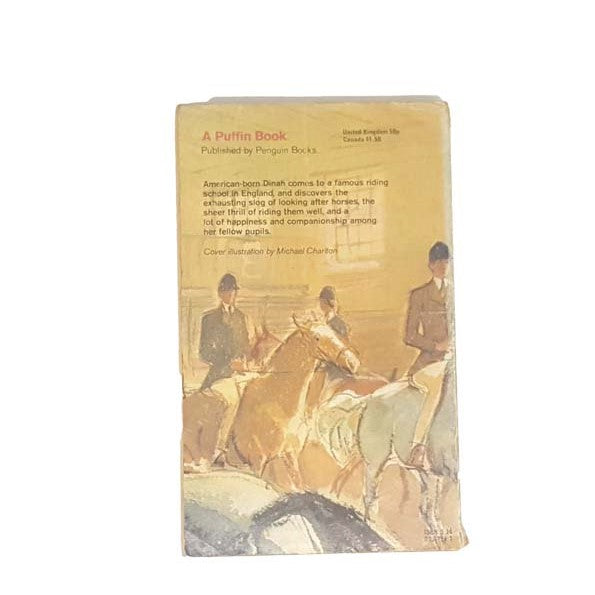This image depicts the back cover of a classic, well-worn book titled "A Puffin Book," published by Penguin Books. The cover, predominantly beige and faded, suggests the book's age and much-loved nature. In bright red letters at the top, it reads "A Puffin Book," with the Penguin Books logo. Below, there's a summary of the story: "American-born Dinah comes to a famous riding school in England and discovers the exhausting slog of looking after horses, the sheer thrill of riding them well, and a lot of happiness and companionship amongst her fellow pupils." The illustrator, Michael Charlton, has depicted three elegantly attired individuals riding on horseback, showcasing a brown and a white horse against a yellowish background. Additional text includes publication details for the United Kingdom and Canada and some accompanying numbers, further emphasizing the back cover's comprehensive information and detailed illustration.